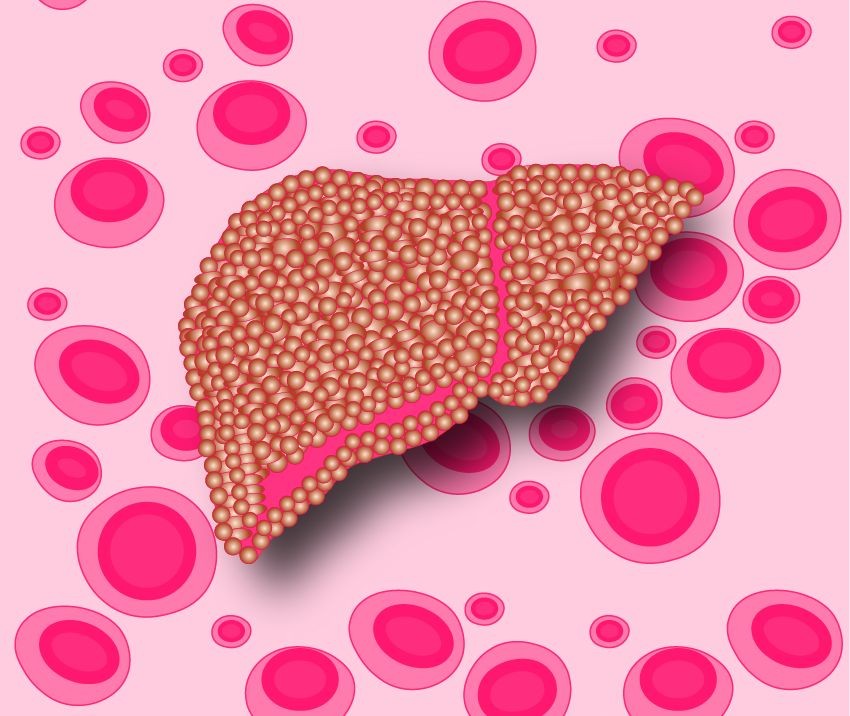The image features a surreal, abstract scene with a dominant central shape resembling a human organ, possibly a liver. This shape is red and pink in color and comprises numerous tiny balls or beads clustered together. These balls exhibit a range of colors including yellow, brown, tan, and burnt pink, with a distinct pattern of white centers transitioning to a darker edge. A prominent hot pink line runs through the middle of this organ-like structure.

Surrounding this central shape, the background is a soft, light pink, populated with various floating circles that evoke the appearance of cells. These circles have pink outlines, with smaller, darker pink centers suggesting red blood cells. The entire composition gives an impression of floating due to the shadow cast beneath the central structure, enhancing the intricate and somewhat medical aesthetic of the scene.